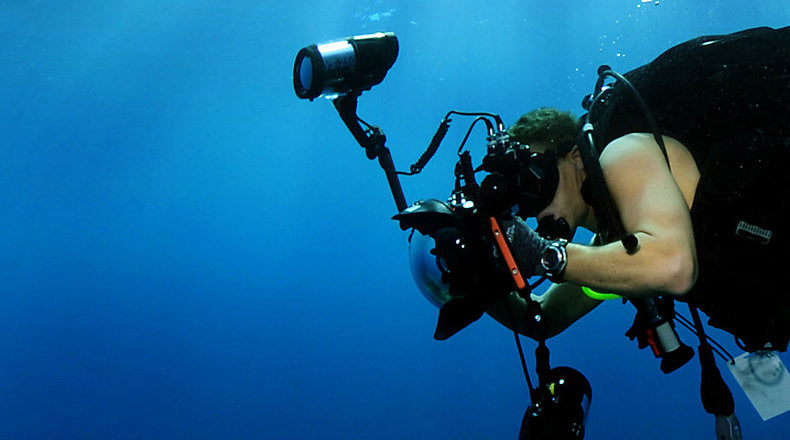In this vivid underwater scene, a determined scuba diver, dressed in a black vest with exposed arms, is captured engrossed in his work. He is outfitted with an elaborate camera system featuring a massive lens and dual lighting attachments, one above and one below the camera. The diver, a strong-looking man with dark hair, is gripping the camera with gloved hands, peering into its large viewfinder, and focusing intently on the seafloor. He is wearing a snorkel in his mouth, a watch on his wrist, and an equipment-laden backpack on his back. The water around him is a rich, deep blue, illuminated by sunlight piercing through the surface, creating a clear, detailed view of the diver and his equipment. The left side of the image is a swath of serene blue, emphasizing the diver's presence on the right side of the frame.